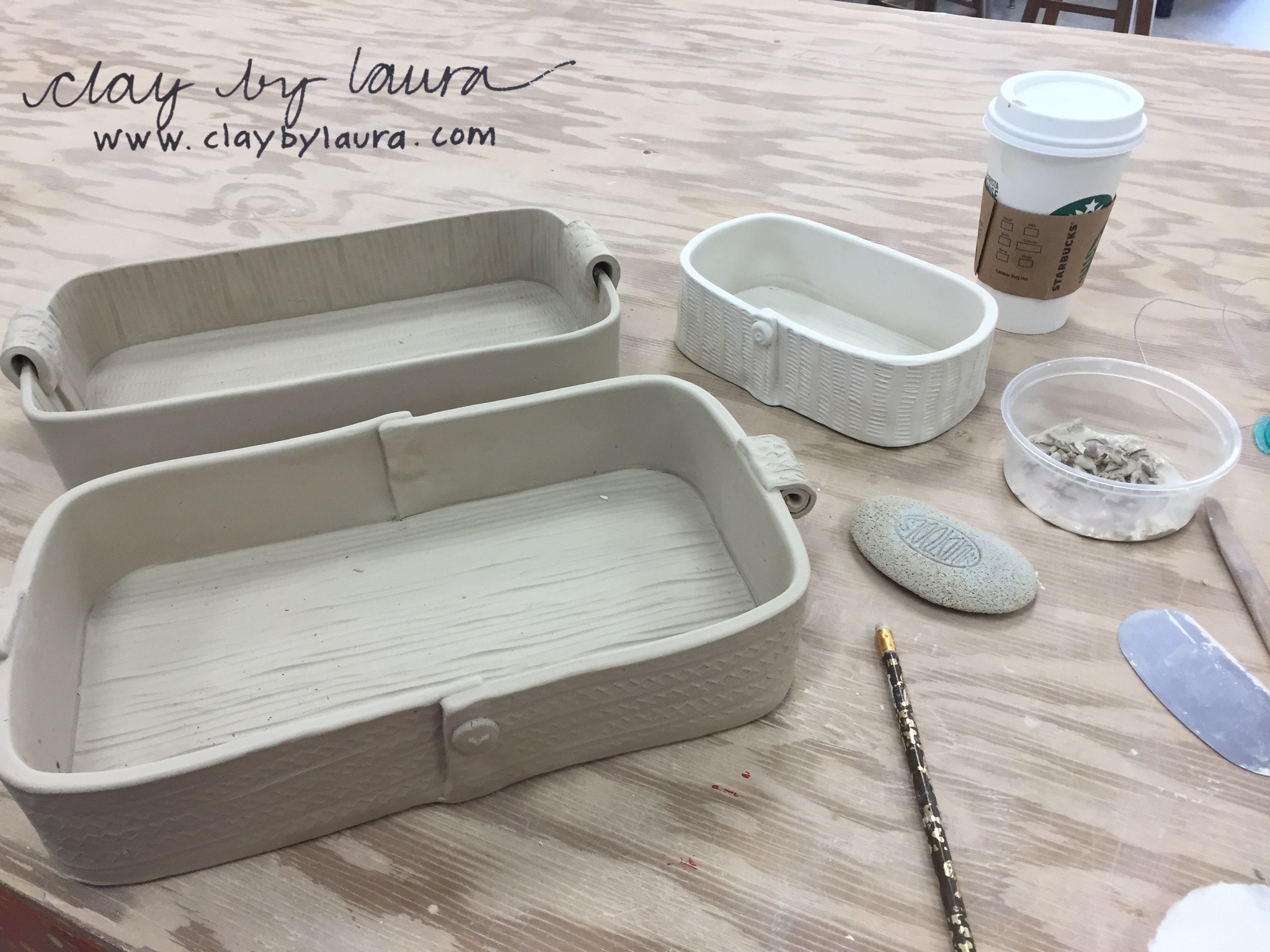The image showcases a promotional setup for a company called Clay by Laura, featuring a detailed and organized wooden table. In the upper left corner, the elegant black cursive script "Clay by Laura" is displayed, accompanied by the business's website, www.claybylaura.com, in a clear print font. On the left side of the table, there are two clay baskets; one is a tan rectangular tray with two handles, and the other is a slightly smaller tray of similar shape. Nestled between these items is a small ceramic container mimicking a wicker design. On the right side of the table, a white wicker basket, which served as an inspiration, stands prominently. There's also a Starbucks coffee cup with a brown recyclable sleeve sitting nearby, suggesting recent use. Scattered across the table are various tools and materials: a disposable plastic dish with clay shavings, a stone with a logo, a wooden stick, a pencil, and a flat scraper — all contributing to the authentic workshop vibe.